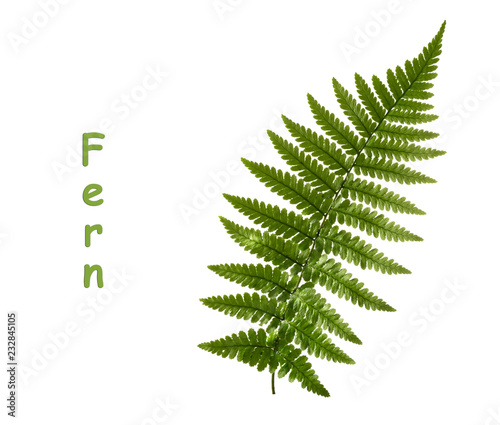The image features a vibrant, healthy fern leaf against a stark white background. The leaf, which is green and composed of a central stalk with similarly structured smaller leaflets on either side, curves gracefully to the right, terminating at a point near the top right of the image. To the left of the fern, the word "FERN" is written vertically in green text, with each letter slightly spaced apart. Further to the left, in small black text rotated counterclockwise by 90 degrees, appears "ADOBE STOCK | #232845105" running from bottom to top along the left side of the image. The composition highlights the lush, well-defined structure of the fern against the minimalistic background.